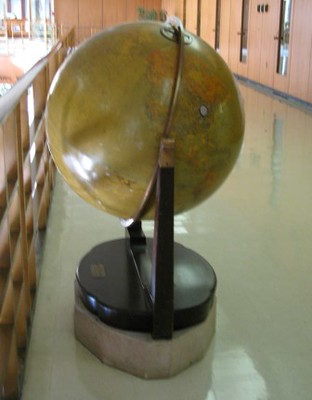The photograph depicts a sizable globe, possibly situated in a school classroom, library, or museum-like setting. This globe, yellowed with age, is prominently displayed in the center of the room, resting on a black pedestal mounted on a sturdy, stone-like white base. The globe, approximately three to four feet in diameter, is noticeably tilted, allowing a clear view of the United States, colored in browns and surrounded by the brown-tinted seas. To its right, Canada is visible in orange, with South America partially obscured by the globe's tilt.

The surrounding environment features a tiled floor and an arrangement resembling a classroom or laboratory. To the left of the globe, there are lab benches with white tops and drawers beneath, while a reddish wood-paneled wall with thin windows and wooden doors forms the background. The opposite wall mirrors this design, incorporating several doors with thin, tall windows. The setting includes additional wooden cabinets and panels, creating a sense of a long hallway or passageway. In the top left corner, a person’s hand reaches out towards the globe, adding a subtle human element to the otherwise static display.